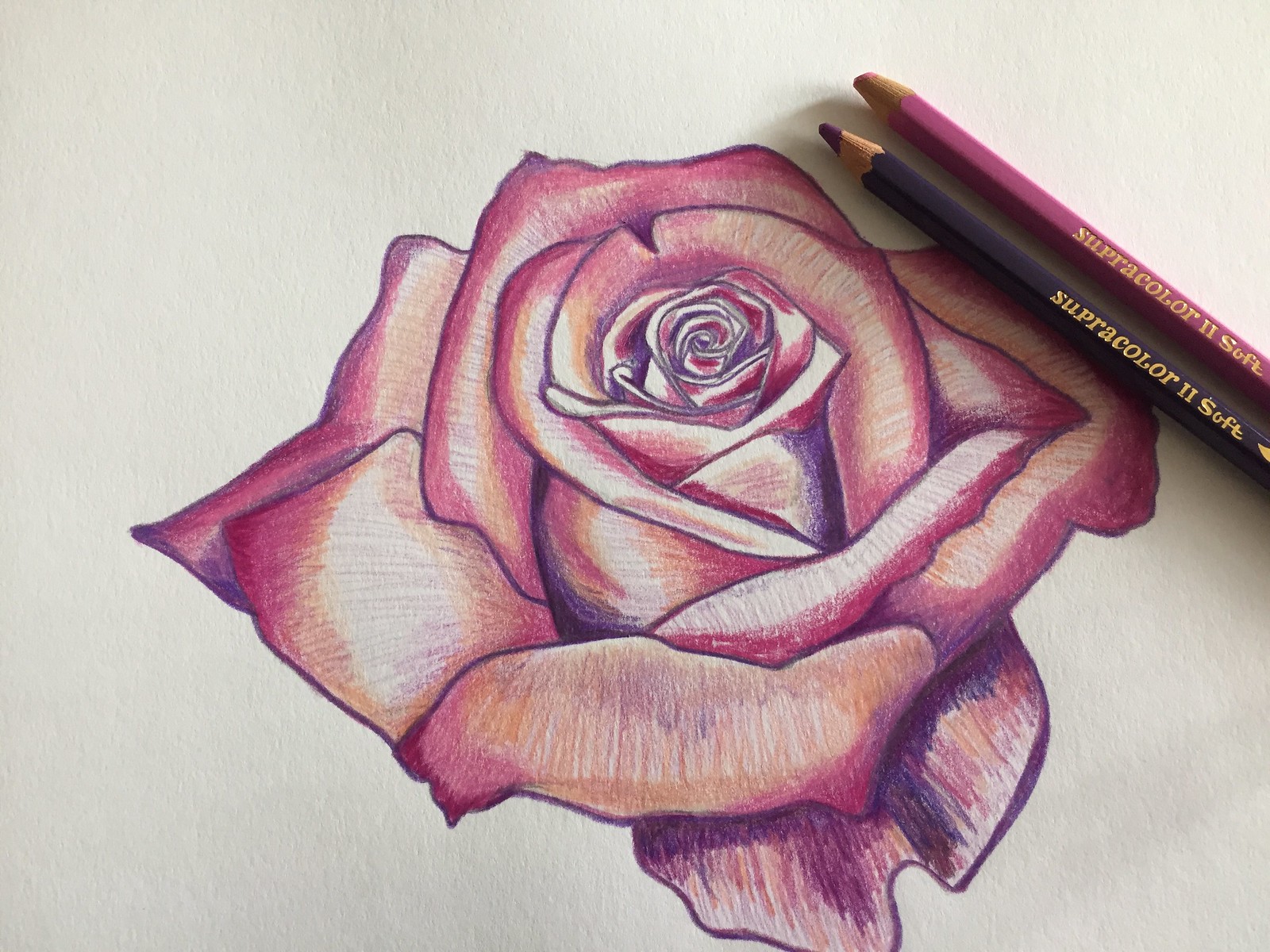This colored pencil sketch features a detailed depiction of a rose bud rendered in varying shades of purple. The artist skillfully applied darker hues at the tip of the bud, gradually transitioning to lighter tones, which include light brownish-orange and white, creating a striking shading effect. Notably, the upper right corner of the composition includes at least two visible pencils, branded as "Supercolor 2 Soft." Interestingly, despite the apparent use of orange tones in the shading, no orange pencil is present in the scene. The sketch exclusively focuses on the rose bud, with no stem or surrounding foliage included.